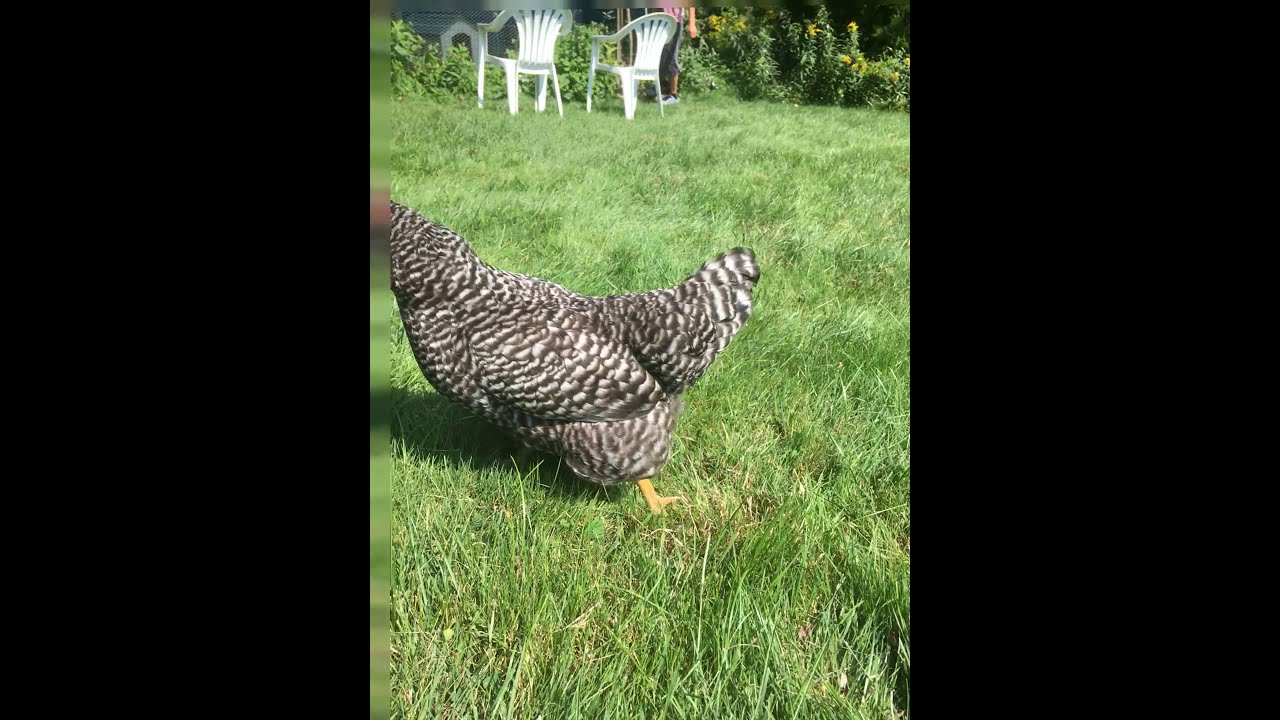This image captures a lively backyard scene dominated by a Plymouth Rock rooster striding across a dense grassy lawn. The rooster's body features a striking mix of dark gray and white speckled feathers, with a vivid red comb partially visible at the top, hinting at its identity. Its sturdy yellow legs are in mid-stride as it appears to be moving swiftly. The chicken's head is unfortunately cut off from the frame, which is bordered on both sides by black rectangles.

In the background, two white plastic outdoor chairs face away, with a person standing nearby, their head out of the frame. The individual is clad in a pink shirt and green or gray pants, partially obstructed by the chairs. Adding a splash of color, yellow flowers with green leaves stand tall behind the person, slightly surpassing the height of the chairs and accentuating the backyard's rustic charm.